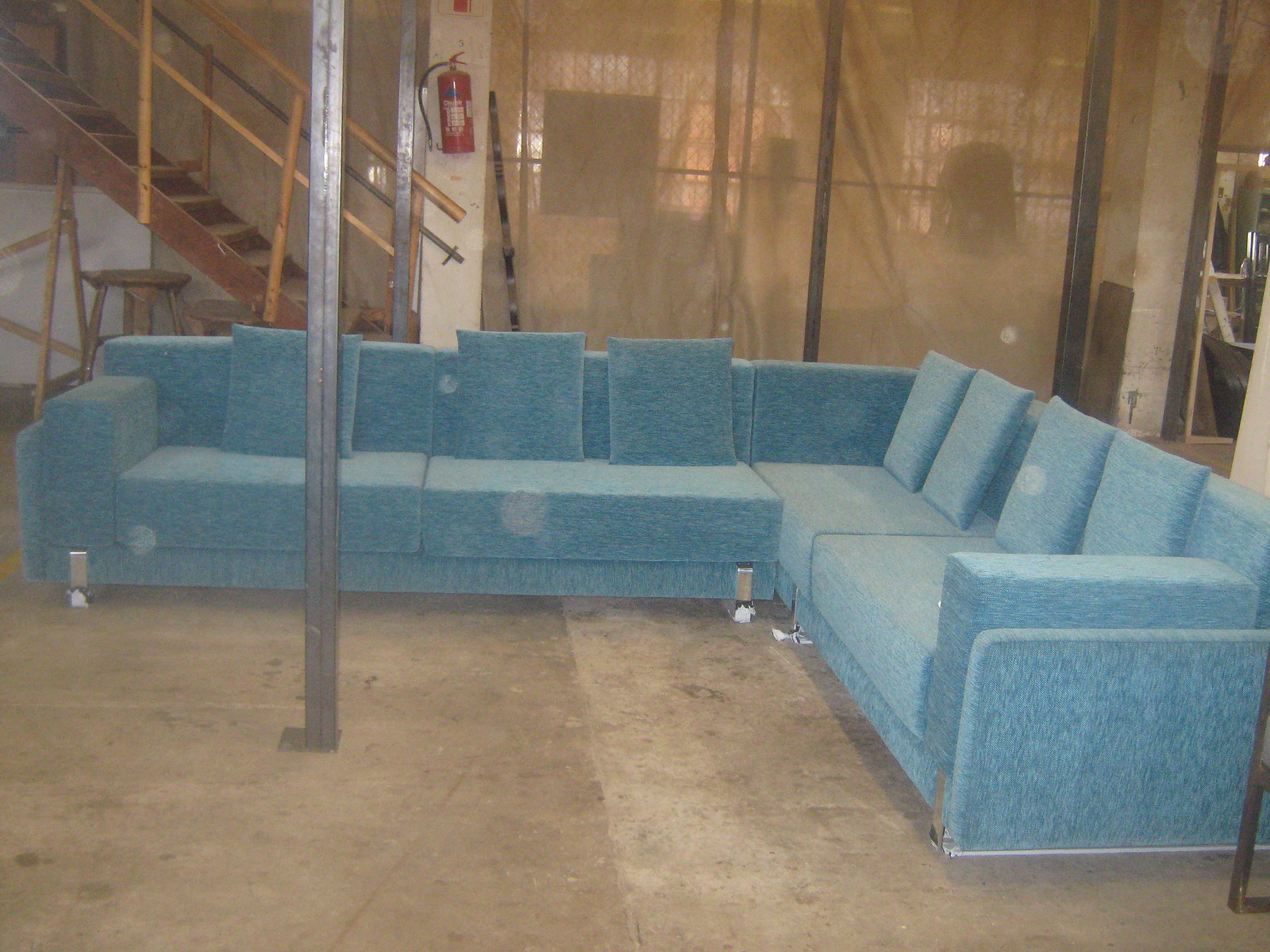In this image, we are viewing a somewhat rundown, unfinished basement living area featuring a large, L-shaped light blue wraparound sectional sofa with a denim-like texture. The sectional, which appears fairly new, has thin, rectangular back supports and numerous flat pillows, resting on thick seat cushions. The basement has a gray cement and possibly unfinished plywood subfloor, and is characterized by exposed structural elements including wooden stairs with thin rails and two brown stools to the left of the staircase. A red fire extinguisher is mounted on the partition wall behind the sofa, next to the stairs. Opposite the fire extinguisher, to the right, is a transparent sheer curtain partially obscuring some windows and other objects behind it. A large black metal beam runs across the room in front of the sofa, and there's an indistinct opening on the far right side, suggesting another area not fully visible in the image.